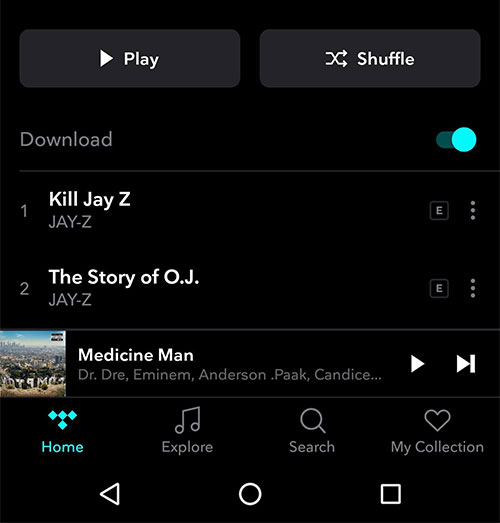A stretched, mobile landscape view of a music app screenshot. The layout features an exaggerated, wide rectangular display, distorting the interface. In the top left corner, large white icons represent the 'Play' and 'Shuffle' buttons, respectively. Directly below, the word "Download" appears in prominent gray text with a toggle switch next to it. The toggle is activated and highlighted in blue.

Underneath, three songs are listed vertically. The third song includes an album cover thumbnail on the left side, accompanied by the song title and artist names in small, gray letters on the right. 

At the bottom of the screen, a navigation bar includes four icons labeled 'Home,' 'Explore,' 'Search,' and 'My Collection'. Beneath this, standard phone interface icons for 'Phone,' 'Back,' 'Home,' and 'Minimize' are visible, completing the layout.